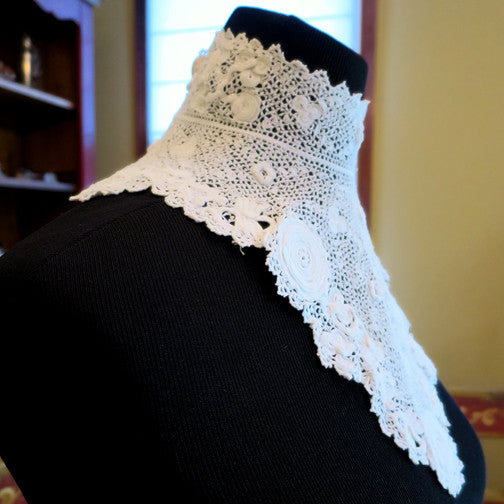The photograph captures the interior of what appears to be a dressmaking shop, with bright yellow walls and a clear window letting in natural daylight. The background features a red cabinet and a bookshelf likely filled with materials. The focal point of the image is a black mannequin torso, velvet-covered and headless, placed prominently in the foreground. Draped over this form is a delicate, off-white, intricately embroidered lace collar. The lace forms a stand-up collar and extends in a V-shape down to the bust, showcasing circles and floral patterns that underscore its Victorian style. The detailed elegance of the collar suggests it is a painstakingly crafted piece, potentially intended for an elaborate, old-fashioned dress.